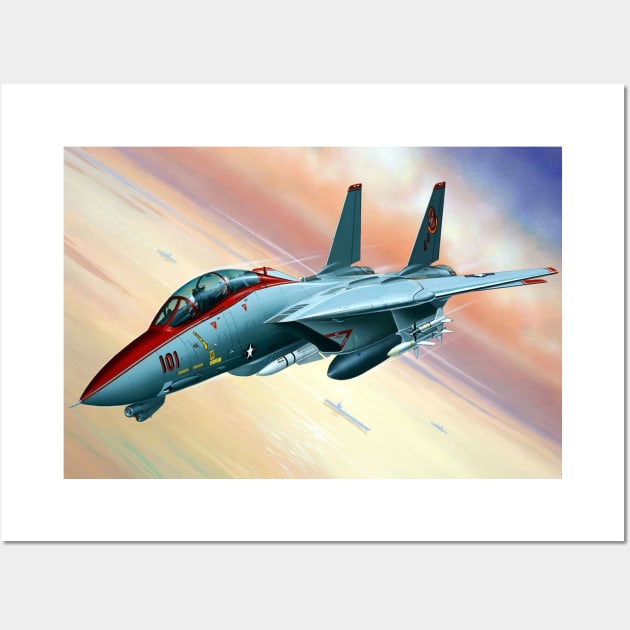The image is a detailed, digitally-generated depiction of a fighter jet, possibly created through painting, drawing, or CGI techniques. The primary colors of the jet are light blue and red, with the front and the border around the main seating area for the pilot being distinctly red. The jet features two rear wings and attached missiles, along with a white star and the number "101" in red text on the side of its body. Inside the cockpit, a figure in a blue outfit, presumably the pilot, can be seen.

The sky in the background forms a colorful, visually striking blend of yellow, pink, orange, light purple, and blue hues, giving it a tilted, surreal appearance. Clouds within the sky contain shades of orange, yellow, and white, and there appears to be a large body of orangey-yellow water visible underneath the clouds, featuring the silhouettes of rowboats. Encasing this vibrant scene is a white border, with the entire composition set against a light gray backdrop. There are no additional texts, numbers, or words visible, apart from the details on the jet. 

Overall, the composition suggests a high level of professionalism and artistic skill, possibly making it suitable for a graphic novel or a video game.